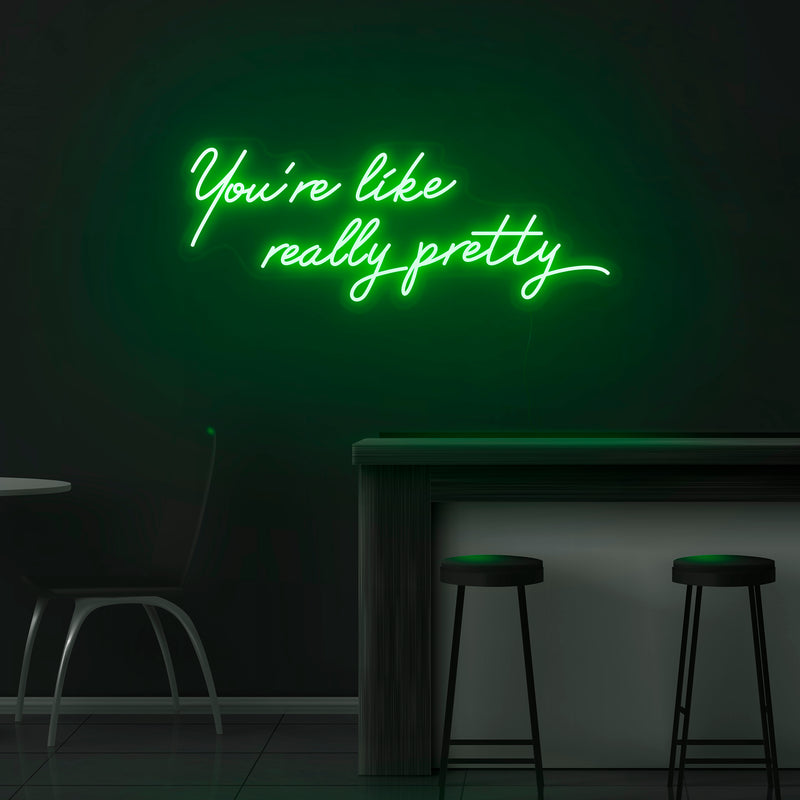In this image, we see a dimly lit bar area with a prominent neon green sign at its center. The script of the sign reads "you're like really pretty," casting a vibrant glow that illuminates the scene. The backdrop of the bar is dominated by a sleek black wall, which accentuates the neon's radiance. To the right, there is a white wooden bar counter with a dark gray top, accompanied by two black bar stools that have dark padding and slightly reflect the green neon light. On the left side, there's a partial view of a white table and a black plastic chair with silver legs. The dark floor below also subtly reflects the neon glow, adding to the room's overall retro ambiance.